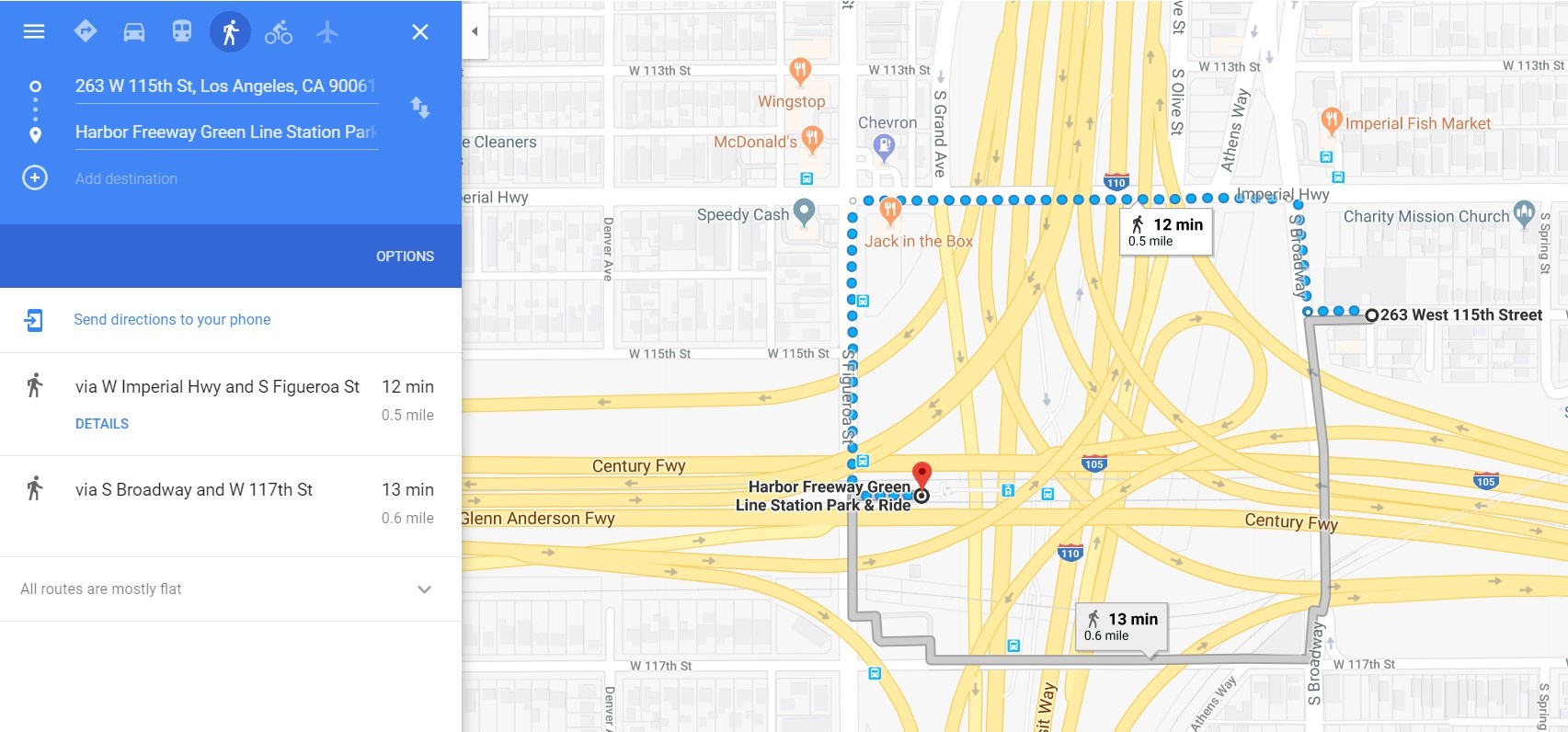A Google Maps screenshot displays a navigational interface featuring a blue dot connected to a gray line, forming a square at the center of the screen. On the left-hand side, various transportation icons are visible, including three horizontal bars (likely the menu icon), a diamond, a car, a bus, a walking person, a bicycle, and an airplane. Additional symbols include an 'X' and a circle. The address "263-W-115-MH, St. Los Angeles, California" is displayed along with a reference to the "Harbor Freeway Green Line Station, PA." Nearby, a circular icon with a dot in the middle appears, along with options for navigating and sending directions to your phone. The suggested routes include: 
1. Via W. Imperial Highway and S. Figueroa Street, taking 12 minutes to cover 0.5 miles.
2. Via S. Broadway and W. 117th Street, taking 13 minutes to cover 0.4 miles.

Both routes are noted as mostly flat.